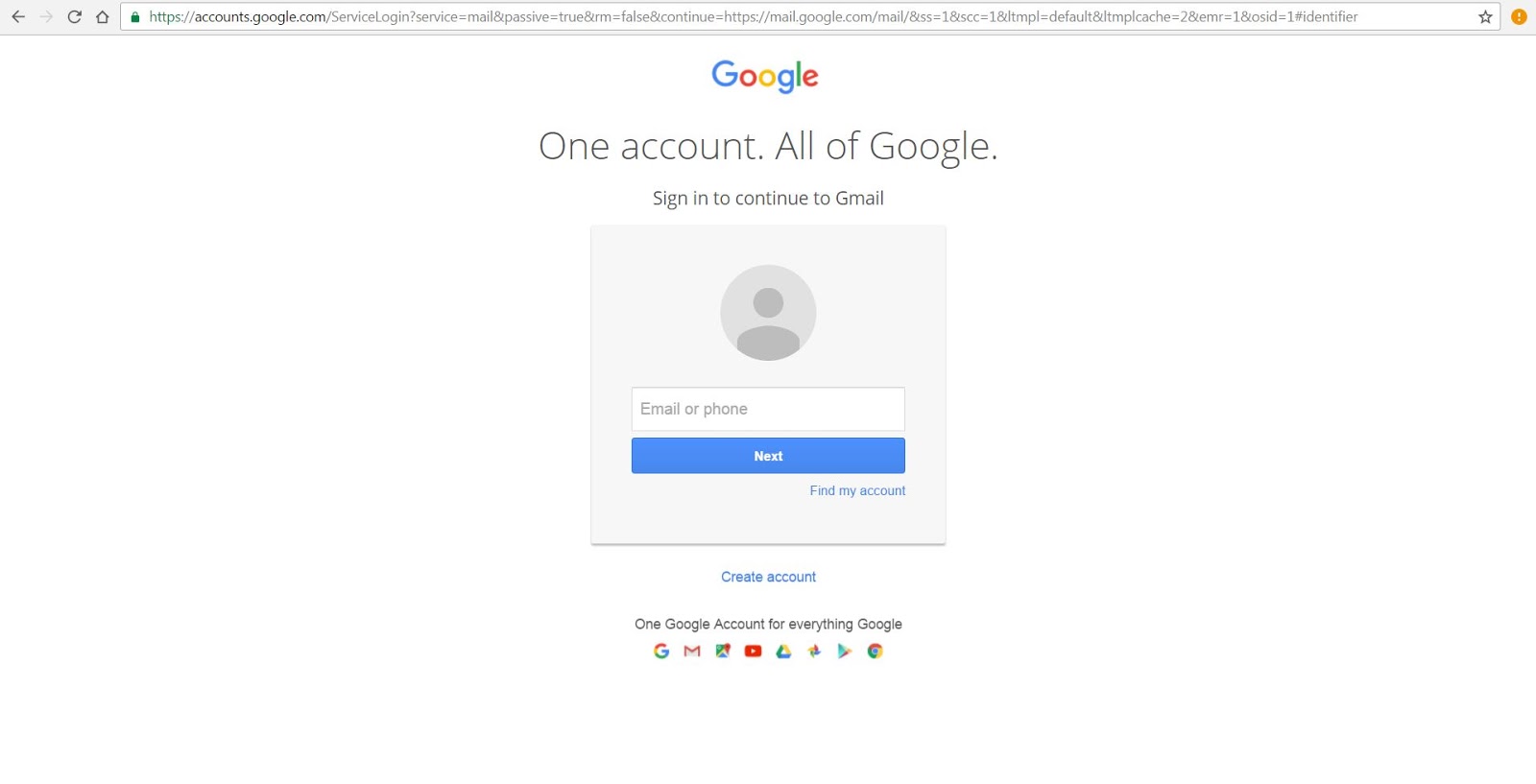The image showcases a Google login page set against a white background. At the top of the page, there is a light blue toolbar featuring a left arrow, refresh and home buttons, followed by a search box. To the right of the search box, there is a star icon and a small orange box with an exclamation point inside. Below the toolbar, the iconic "Google" logo is prominently displayed with its familiar blue "G," red "O," yellow "O," blue "G," green "L," and red "E."

The text beneath the logo reads, "One account. All of Google. Sign in to continue to Gmail." Directly under this statement is a blue box with a circle containing a person icon, symbolizing user identification. There is an input field labeled "Email or phone," followed by a blue "Next" button which includes the additional text "Find my account."

Further down the page, there is an option to "Create account." Near the bottom of the image, it states, "One Google Account for everything Google," accompanied by recognizable icons for Google services such as Mail and more.